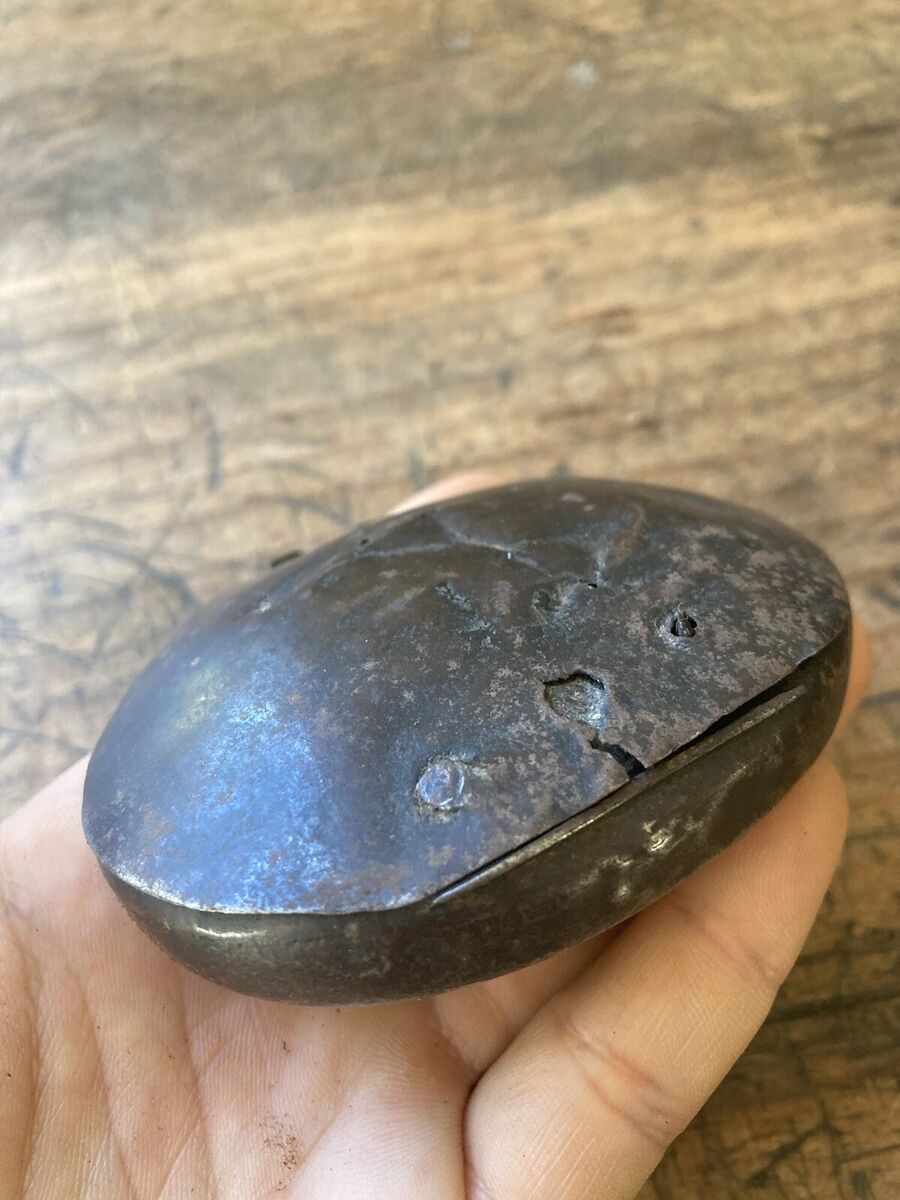An up-close photograph captures a fair-skinned human left hand holding an ancient, dark gray metallic box with a lid, potentially resembling an artifact found at an archaeological site. The hand is positioned over a worn wooden table, characterized by deep scratches, a light tan hue, and gray markings. The hand's pinky finger is visible, while the other fingers are obscured by the box. The metallic box, exhibiting significant deterioration at the edges, features cracks and lighter gray splotches on the surface. Notably, the front of the box has a distinct white pattern with a central spot, and a line where the two halves would separate. The box might also serve as a container, suggested by a small rectangular notch at the back, resembling a hinge. The base of the box is oval, and the lid does not sit flush with the base, revealing gaps. Despite its rough, primitive appearance, and signs of wear and broken mechanisms, the box carries an ornate quality, hinting at its ancient and possibly utilitarian origin.